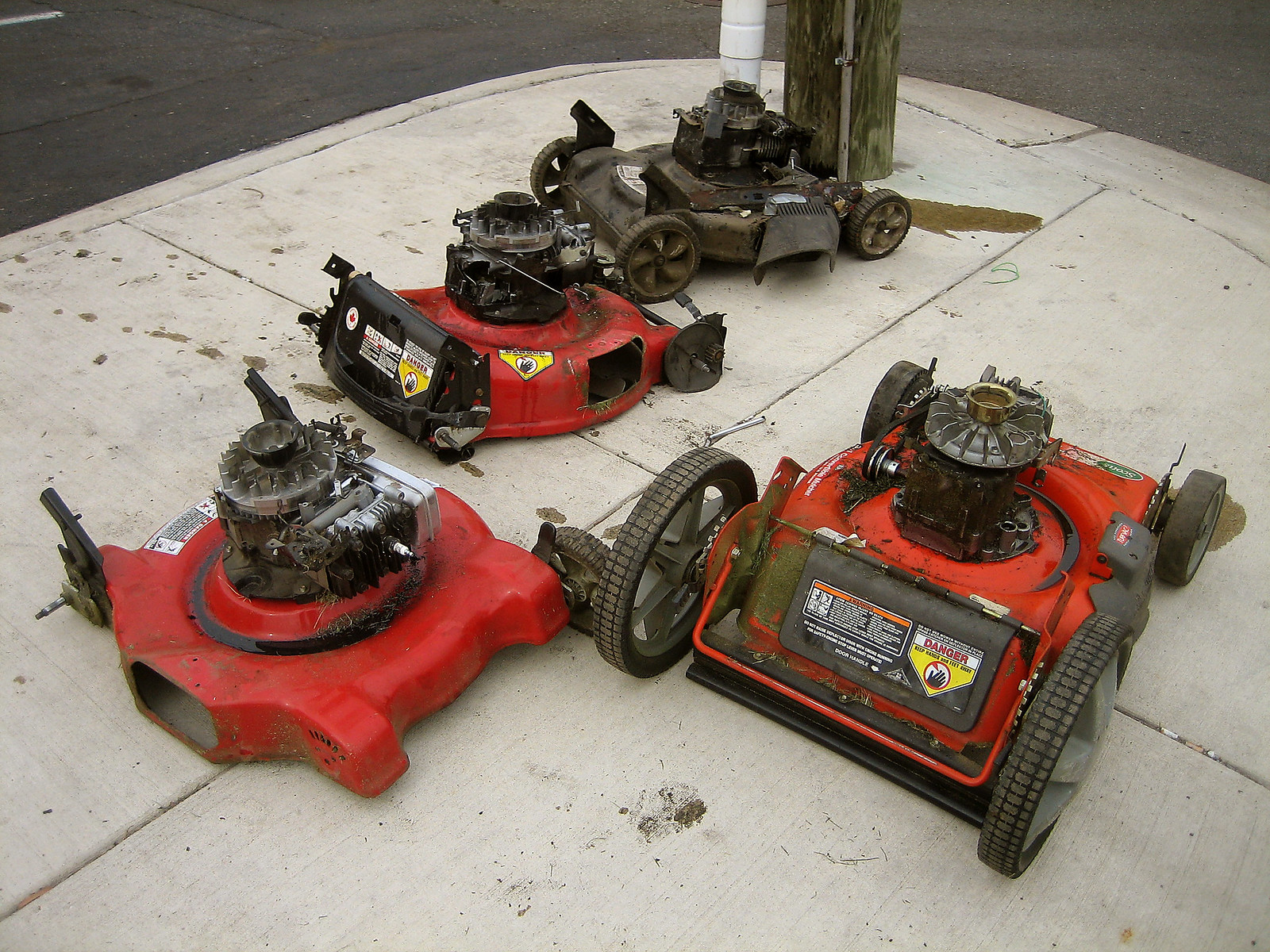The image depicts four hand-pushed lawnmower bodies without handles, positioned on a light gray sidewalk at the corner of two streets. In the background, a dark gray road and a wooden telephone pole or power pole can be seen, along with a white pipe. On the left-hand side of the image, there are three similarly sized lawnmowers; two have red bodies and are missing all their wheels, while a dark green mower appears to have at least three wheels, though the fourth is obscured. On the right-hand side, there is a larger red lawnmower with bigger wheels, all of which are intact. The engines of the mowers are exposed, and the overall scene conveys an odd placement of these lawnmower parts on the sidewalk, raising questions about why they are there.